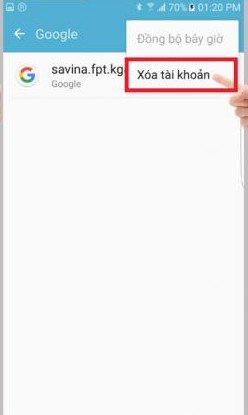The image presents a partial view of a smartphone screen. The top of the screen displays typical status icons including a computer signal, a 70% battery indicator, the time (1:20 PM), and network strength. There is a back arrow pointing to "Google," suggesting a return to a previous screen. Below this, a blue banner spans the top, encapsulating these icons.

Centrally, the screen shows a single Google search result. The link in this result reads "savina.fpt.kg." Adjacent to this link, a red-highlighted phrase, "xoá tài khoản" (likely Vietnamese), is emphasized by a pointing finger icon. Above this, a faded rectangular overlay in a shade of gray contains the text "Dong Bo Bai Zhou," though the meaning is not clear. The red highlight and the emphasized Vietnamese phrase appear significant but their exact context or translation is not provided.